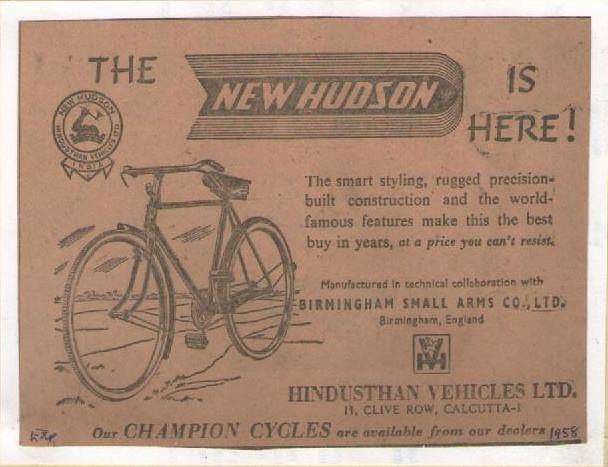This image depicts a vintage 1958 advertisement for a bicycle, set against a mottled beige-brown background that resembles old, faded newspaper or cardboard. Dominating the top left is a small logo beside the bold proclamation, "The New Hudson is here!" This is accompanied by a stylized arrow symbol featuring the phrase "NEW HUDSON." The text beneath enthusiastically highlights "The smart styling, rugged precision-built construction, and world-famous features make this the best buy in years at a price you can't resist."

To the left of the text, there is an illustration of a vintage 10-speed bicycle with flat handlebars, rod brakes, and double fenders, depicted idly against a sketched backdrop that resembles a countryside roadway. Below the image, the advertisement notes the manufacturing collaboration with Birmingham Small Arms Company Limited, Birmingham, England. The bike is distributed by Hindustan Vehicles Limited, located at 11 Clive Row, Calcutta. The bottom of the ad assures potential buyers, "Our champion cycles are available from our dealers," with "1958" clearly marked in the bottom right corner.